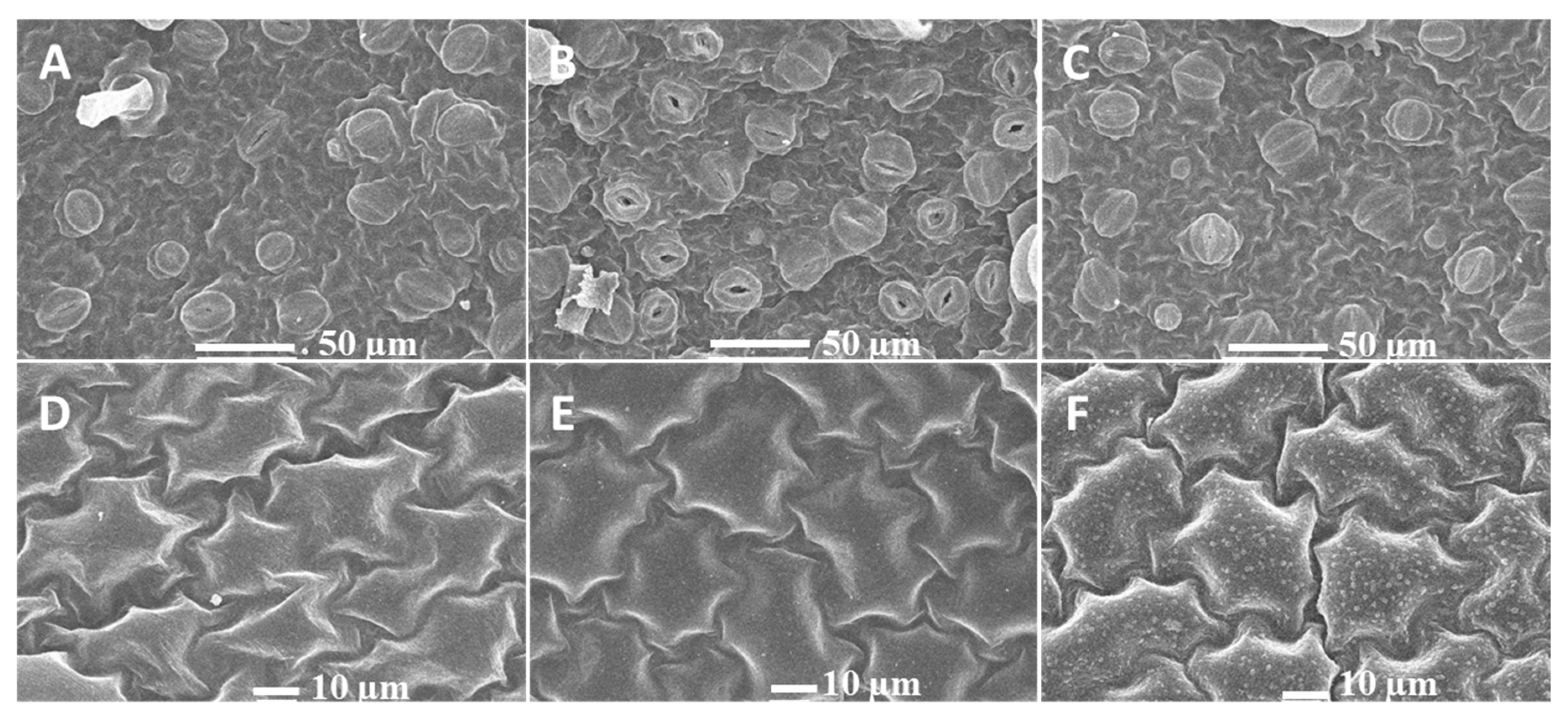This image is a six-part scanning electron microscope presentation focused on gene and metabolite integration in relation to heat stress tolerance in potatoes (Solanum tuberosum). The image comprises six grayscale pictures labeled A through F, each displaying a different magnification of potato cells. 

The top row, consisting of images A, B, and C, has a scale bar marked "50 µm," indicating a zoomed-out view. In image A, the cells are solid gray shapes. Image B shows similar shapes with some black holes appearing within the structures. By image C, the shapes have fewer clusters and display some white lines running through them.

The bottom row, containing images D, E, and F, is further magnified with a scale bar marked "10 µm," showing a more detailed view. Here, the cellular clusters transform into rigid, circular forms with sharp, pointy edges, connected together. Image F is distinguished by the presence of numerous small white spots scattered over these shapes.

Across all images, the shift from the less magnified top row to the more magnified bottom row reveals increasingly detailed structural features and variations in cellular formation under heat stress, providing a comprehensive view of cellular responses at different scales.